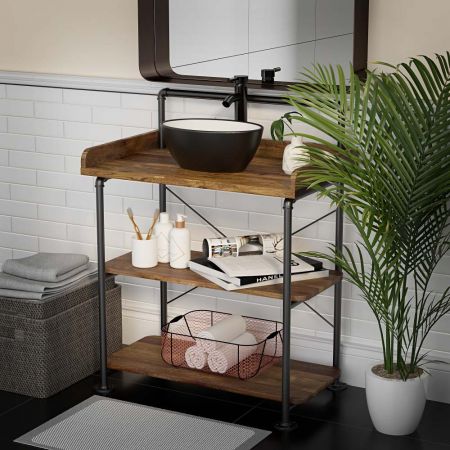This photograph captures a clean and stylish bathroom with several distinct features. Central to the image is a unique vanity designed more like a shelf, constructed from wood and metal pipes. Atop this vanity sits a sleek black water bowl-style sink and faucet. Adjacent to the faucet, the wooden vanity holds white containers for toothbrushes and soap, flanked by magazines. Below, the lower level of the vanity shelf houses a gray crochet-patterned canister containing neatly rolled white towels.

The background showcases an attractive white brick tile that climbs up to the cream-colored upper portion of the wall, where a mirror is situated, reflecting the tiled wall below. To the right of the vanity, a vibrant green indoor plant in a white base adds a touch of nature. On the left, a storage compartment holds more towels, while a mat rests on the black flooring in front of the entire setup. The thoughtfully arranged elements and materials create a harmonious and inviting bathroom space.